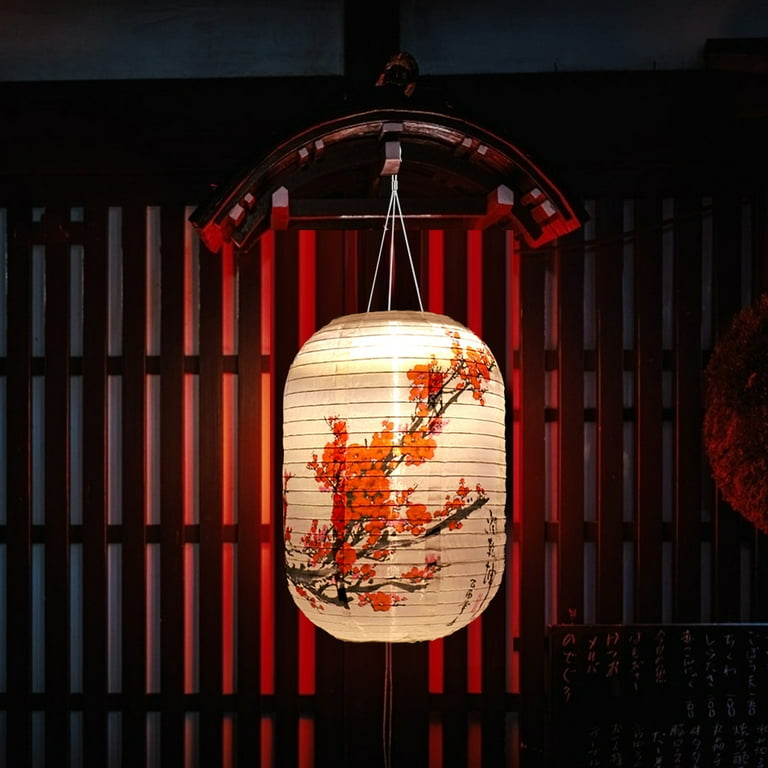The image depicts an ornate, oval-shaped Asian lantern, likely Japanese or Chinese in origin, hanging gracefully from a wooden arch or post attached to the ceiling. The lantern itself is primarily white and adorned with a striking design of reddish cherry blossoms on dark branches. Some Japanese lettering is visible on the bottom right of the lantern. The background features a wall made of dark wood planks, adding to the ambiance. The scene is set in a predominantly dark environment, with the glow of the lantern casting a warm, yellowish light that highlights its painted flowers and illuminates the immediate area. The outer edges of the image remain in shadow, creating a dramatic vignette effect. Additional lighting in the background hints at a red-hued wall or structure, further enhancing the rich, atmospheric setting.